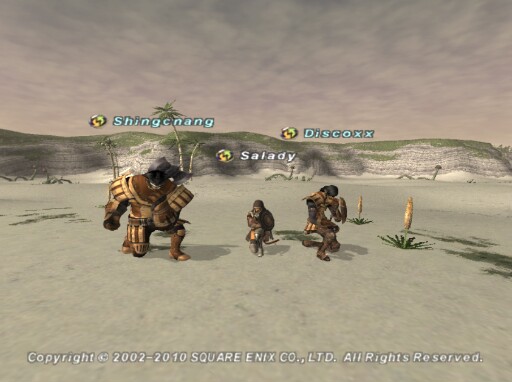This screenshot is from a video game, capturing a moment set in the middle of a vast desert. The scene features three distinct characters whose names are displayed above them. On the left stands an enormous character with hooved feet, its face obscured and angled downward; the name “Xing Chang” hovers above in white text. In the center is a diminutive figure, appearing in a shade of brown with scarce visible details, labeled “Salady” in white. To the right is a character kneeling, head bowed, clad in a brown leather outfit, with black hair, named “Disco X” in blue text. The desert ground is a stark white sand, contrasting against the backdrop of hilltops adorned with grass, their sides remaining sandy. A copyright notice stretches across the bottom of the image, reading: “Copyright 2002-2010 Square Enix Co., Ltd. All rights reserved.”